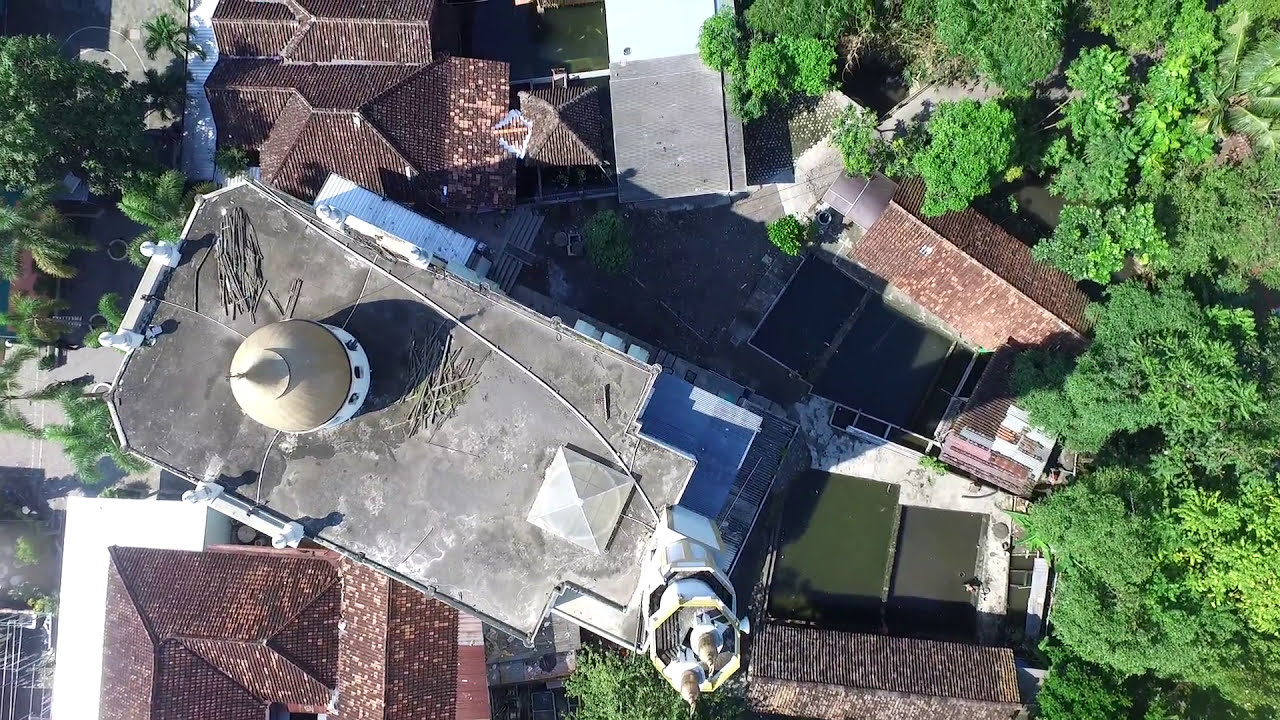This detailed aerial photograph, taken during the daytime, provides a nearly vertical view of a complex of buildings. Dominating the center is a large, flat-roofed building with a distinct dome-like steeple that is brown with a pointed tip, possibly resembling a rotunda with a spiral roof. The roof of this central building appears to be constructed from a brownish stone or concrete slab, and scattered across it are various items including wooden planks and metal poles. To the right edge of this building’s roof, an air conditioning unit is visible.

Surrounding this central structure are several older buildings with traditional sloped roofs, covered in worn red, brown, and white tiles. The layout of the buildings appears to create a small complex interconnected by concrete walking paths. To the far right and left sides of the image, dense clusters of trees, including palm trees, are present, offering some greenery. Among these trees are more sparsely arranged trees, adding to the lush surroundings.

Additionally, the bottom left of the image hints at possibly a covered pool area, suggesting recreational facilities within the complex. The rooftops, trees, and walking paths collectively suggest this might be a residential area, potentially with multiple homes sharing communal spaces. The arrangement and details of the photograph provide a comprehensive view of the surroundings, blending the natural elements with the architectural features of the buildings.